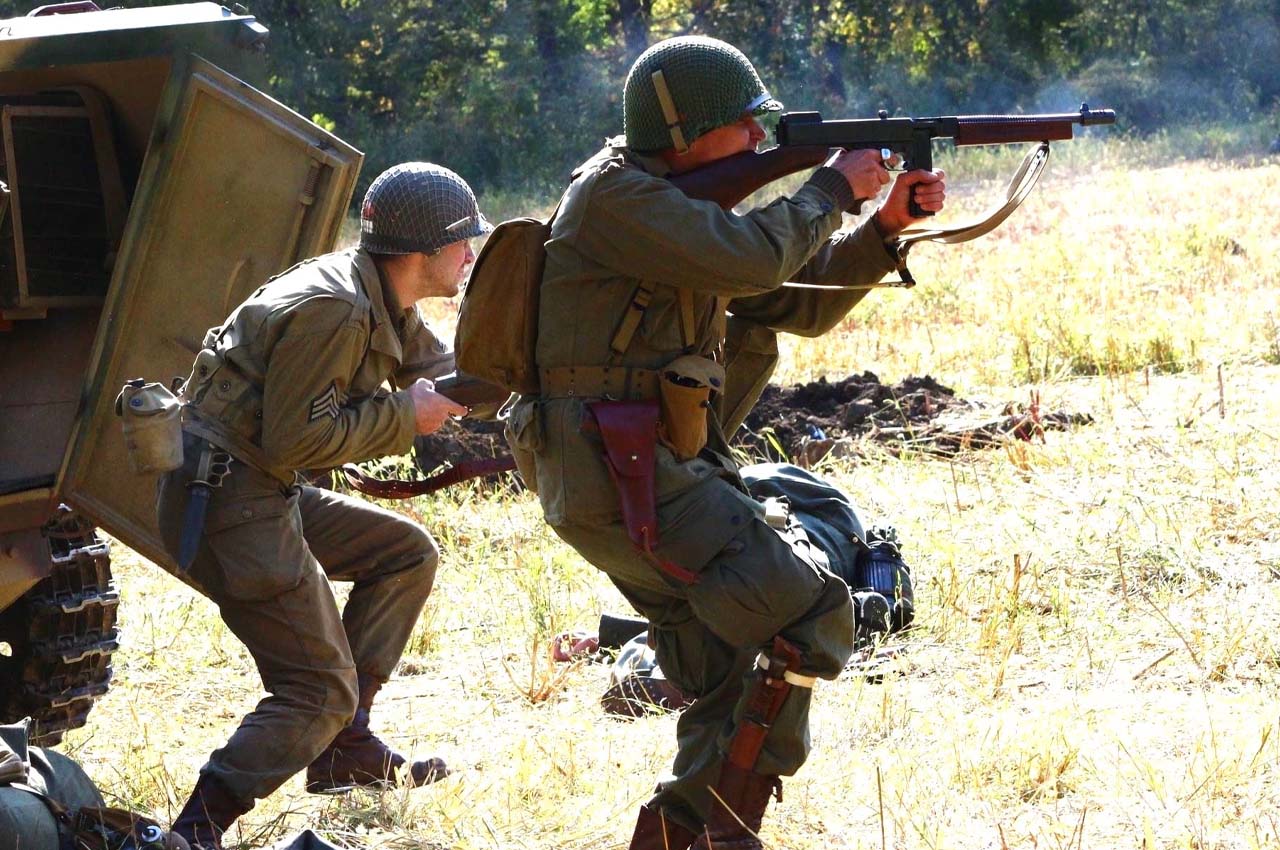In a high-exposure photograph, two soldiers are captured in the midst of combat, emerging from an olive green military vehicle with its door open and treads visible. Both soldiers are dressed in dark, olive green tactical gear with rounded helmets and brown boots. The soldier on the right is aiming a rifle, with additional gear including a yellow pouch on his shoulder and a red holster. A knife and sheath are attached to his boot. The left soldier, holding a rifle in both hands, has a knife strapped to his belt next to a canteen and three white triangle patches on his attire. They are standing in an open field with nearly white grass due to the high exposure, and there is a faint squash yellow hue permeating the scene. A figure lies on the ground nearby, possibly injured or deceased. In the background, shrubbery and trees emerge through a delicate layer of light fog, adding a sense of depth and tension to the moment.